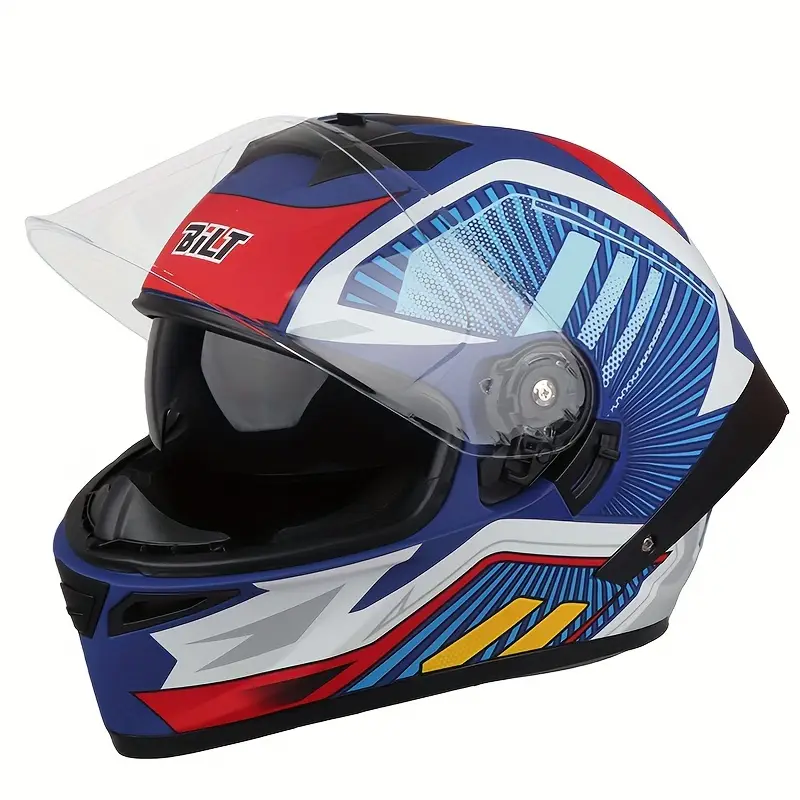The image depicts a vibrant motorcycle helmet featuring a comic book-inspired design with multicolored patterns. The helmet predominantly showcases blue sections, complemented by red and yellow streaks, and white stripes and dots around the ears and jawline. Noteworthy is the manufacturer's name, "BILT," prominently displayed at the top, with black letters outlined in white and a red dot on the "I". The helmet also includes various white, light blue, and rectangular shapes that contribute to its dynamic appearance. The interior is lined with black padded leather for comfort, and it features a clear, flip-up visor that protects the eyes. Additionally, airflow vents are incorporated into the design, providing top and front ventilation. A black cloth strap ensures the helmet stays securely fastened. The helmet is facing left, with the back visible to the right.